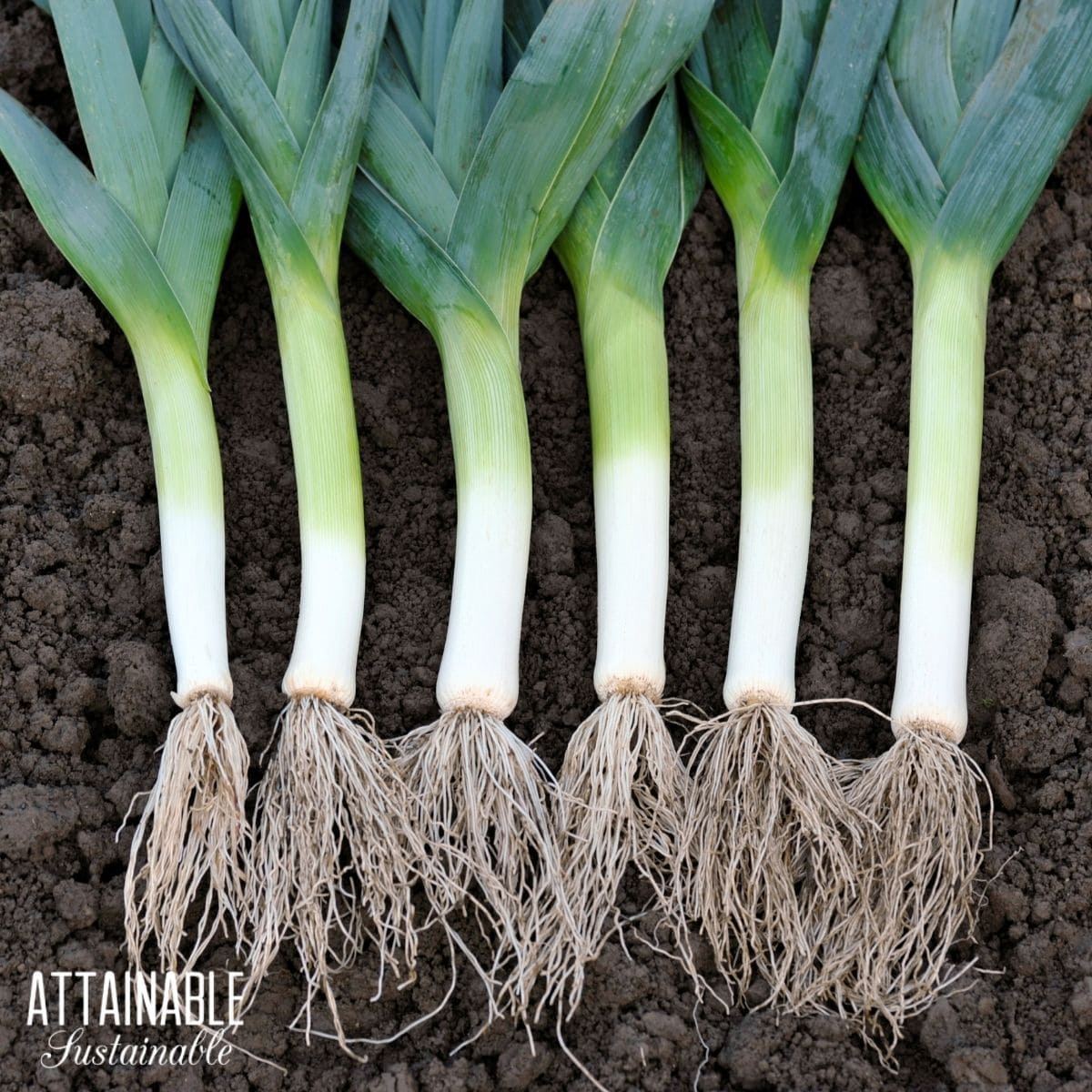In the image, six large leeks are freshly dug up from the dark brown, almost blackish, loose soil. The leeks are arranged horizontally across the middle of the frame, their long, hairy-looking roots prominently displayed at the bottom. The plants feature a white stem transitioning into a light green shaft, which further develops into broad, dark green leafy tops, though the tops are cut off about two inches up, not showing the entire plant. The soil underneath and around the leeks is notably dark and loose, forming a contrasting background. In the bottom left corner of the image, in white capital letters, it reads "ATTTAINABLE," and just below in cursive, "SUSTAINABLE." The vibrant colors of the leeks, ranging from white to various shades of green, stand out against the rich dark soil. The clean appearance of the leeks suggests they have been freshly harvested.